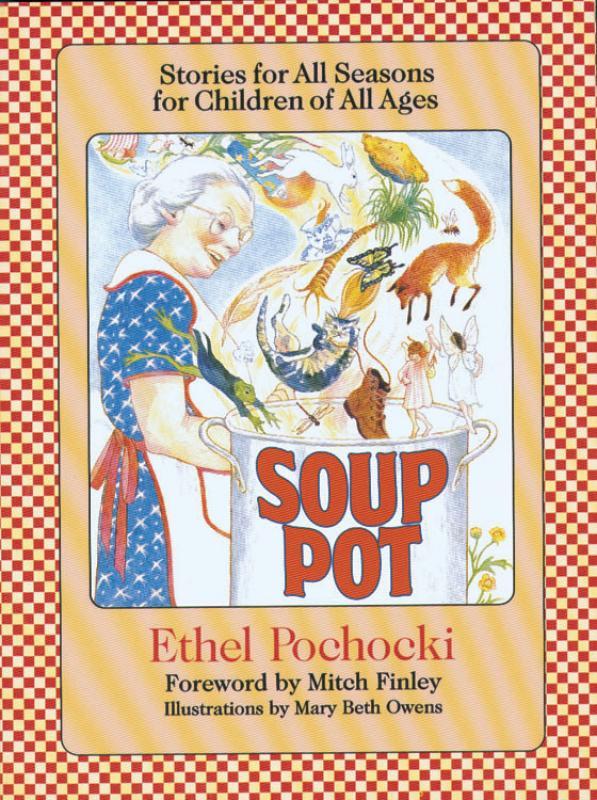The book cover features a vibrant and whimsical design, bordered by a striking red and white checkerboard pattern. Inside the border, the background transitions into a warm, yellow and pinkish hue with subtle gold stripes, all meticulously outlined in black. At the top, the bold, black text reads, "Stories for All Seasons for Children of All Ages."

Dominating the center of the cover is a charming illustration of an elderly woman with silver hair, dressed in a blue dress with a white and red apron. She appears intent on making soup in a large, silver stock pot labeled "Soup Pot" in prominent red letters. Surrounding her are an eclectic mix of items appearing to be tossed into the pot: a cat, a shoe, little fairies, a fox, a butterfly, various roots, and even an entire pie. 

Below the illustration, the author's name, "Ethel Pochocki," is displayed in red letters, followed by the text "Foreword by Mitch Finley" and "Illustrations by Mary Beth Owens" in black. The overall scene encapsulates an enchanting and playful aesthetic, inviting readers into the delightful stories within.